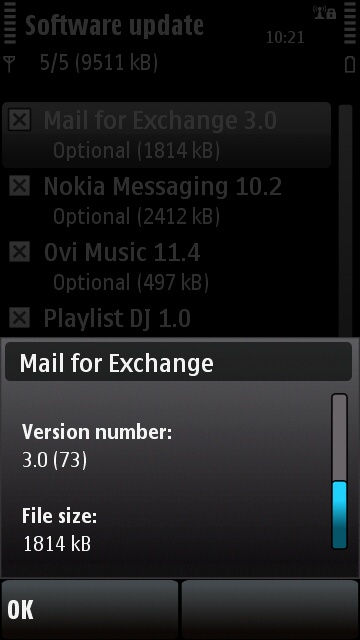In this image, there is a smartphone screen showing a software update notification, set against a black background. The image is very blurry and distant, making the details hard to discern. The notification indicates a software update version 55, with a file size shown in parentheses as (9511 kilobytes). The screen display reads the time as 10:21. 

The update details several optional components, each marked with a small "X" to indicate they can be excluded:
- Mail for Exchange 3.0 (1814 KB)
- Nokia Messaging 10.2 (2412 KB)
- Ovi Music 11.4 (497 KB)
- Playlist DJ 1.0

Below the main notification, there is more specific information about the "Mail for Exchange" feature:
- Version number: 3.0
- File size: 1814 KB

To the right, there is a long button that is black at the top and light blue at the bottom. At the bottom of the screen, there are two smaller buttons. The left button has "OK" printed in white, and the right button is blank.